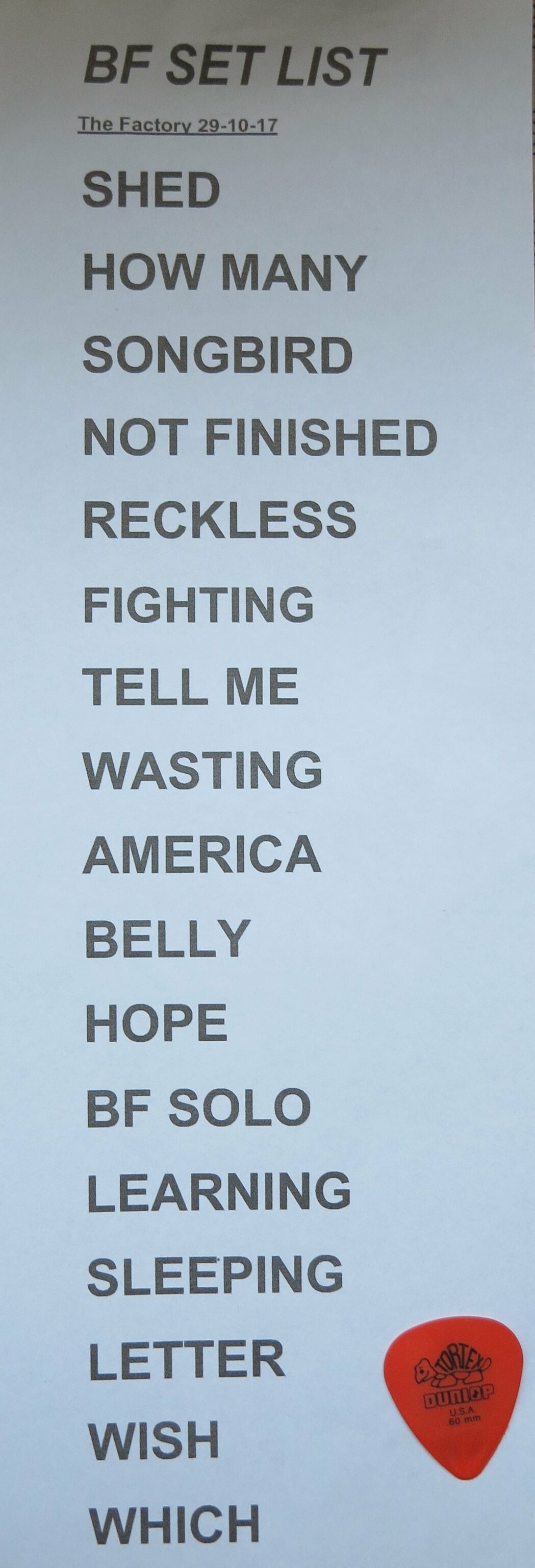The image depicts a light bluish background featuring a long piece of paper with a list of words. At the top of the list, in black font, it reads "BF setlist," followed by "the factory 29-10-17," possibly indicating the date and venue. The list continues vertically with the following entries: "shed, how many, songbird, not finished, reckless, fighting, tell me, wasting, America, belly, hope, BF solo, learning, sleeping, letter, wish, which." In the bottom right corner of the image, there is a red guitar pick adorned with a cartoon image of a turtle. The guitar pick is labeled with "Dunlop" beneath the turtle, indicating it is a Dunlop guitar pick. This creates the impression that the image showcases a band's setlist along with a significant musical accessory.